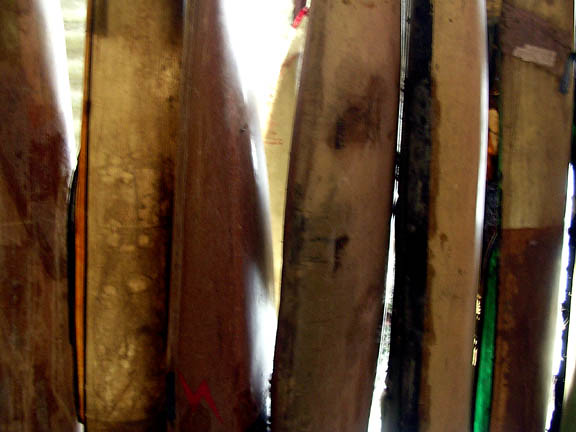This colour photograph captures a close-up view of various vertical wooden objects that span the entire frame, both vertically and horizontally. Due to the image's proximity, the objects are slightly out of focus, making it challenging to identify their true nature. At first glance, the objects resemble badly designed vertical fence posts, but upon closer inspection, they seem to have a slight curvature suggestive of wooden surfboards, or possibly parts of a fence. The materials vary in colour and texture, with some pieces being a lighter pinkish wood and others a darker, reddish oak. There is evident wear and weathering, with some showing dark markings and even black bark on the side. Additionally, a piece on the far right features a green line, and another near the center has a red lightning bolt design. The objects are unevenly leaning against each other, and sunlight pierces through the gaps, casting bright light between them. Despite the unclear view, elements like a bit of stairs and a yellow object are partially visible behind the wooden array, adding to the mystery of their purpose.